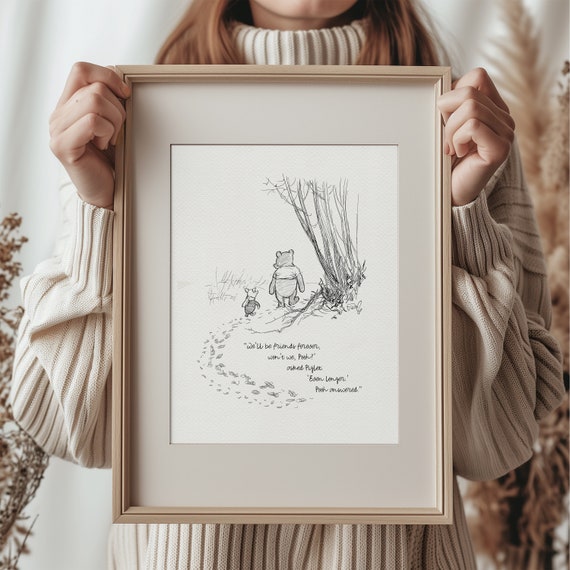In this color photograph, a woman with long, reddish-brown hair is holding a framed illustration from the British Winnie the Pooh novel. The drawing, encased in a light brown wooden frame with a light gray mat, depicts Winnie the Pooh and Piglet walking in the snow, their backs to the viewer, with footprints trailing behind them. Trees are visible on the right side of the image, adding to the wintry scene. The illustration features black, handwritten text that, while mostly blurred and difficult to read, includes the quote: "We'll be friends forever, won't we Pooh? Asked Piglet." Below the quote, additional smaller text is present but unreadable.

The woman, dressed in a light beige, cable knit, ribbed turtleneck sweater, holds the picture frame on either side, but her face is not visible in the frame. The focus is solely on her hands and the charming illustration she presents.